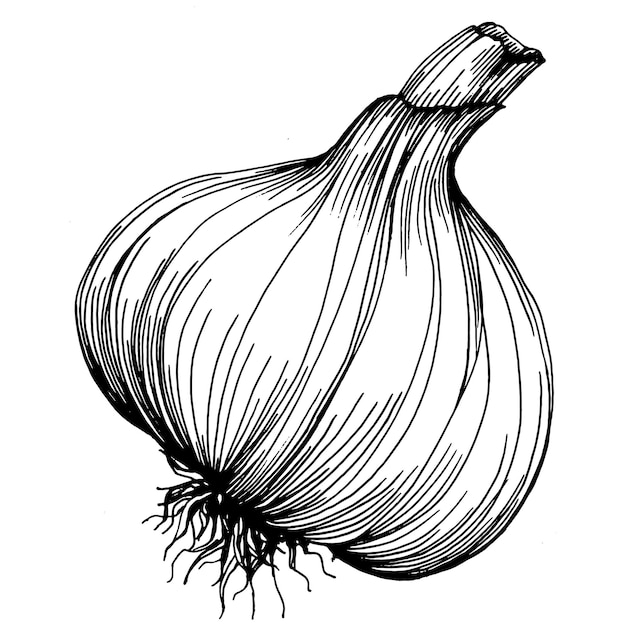This is a detailed black and white line art drawing of an unpeeled onion, centered on a white background. The onion, which has an oval-like shape and is oriented with its roots facing the bottom left corner and its stem extending towards the top right, is depicted with intricate line work. The image showcases the onion's layers and the realistic, hair-like roots at the bottom. The stem, extending from the top, is also detailed with numerous lines that capture the essence of its texture. Despite the lack of shading or background elements, the multiple lines running vertically around the onion provide a distinctive sense of depth and detail, making it appear as though it could be a piece that someone might color in. The meticulous depiction includes detailed roots and layered skin, emphasizing the natural complexity of the onion.